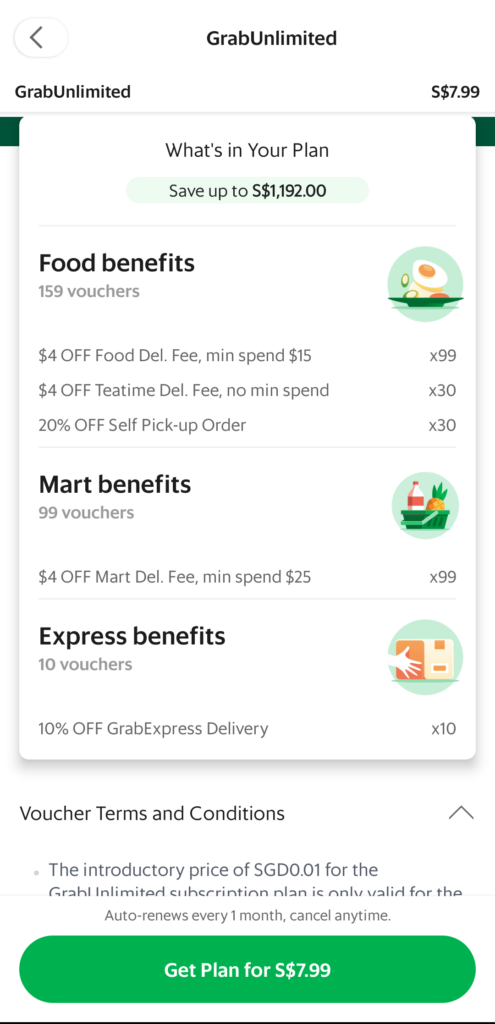This screenshot displays the Grab Unlimited subscription plan from a mobile application. The interface prominently features "Grab Unlimited" at the top and on the left side. The subscription cost is clearly listed at $7.99. The plan highlights significant savings, claiming users can "save up to $1,192" through various benefits.

Under "Food Benefits," the plan offers $159 in vouchers, divided into three types. Next, under "Market Benefits," there are $99 in vouchers. Lastly, "Express Benefits" provide $10 in vouchers. Below these details, there's a section titled “Voucher Terms and Conditions” with an expandable arrow for more information, followed by text indicating the plan auto-renews monthly and can be canceled at any time. At the bottom, a prominent green button encourages users to "Get Plan for $7.99."